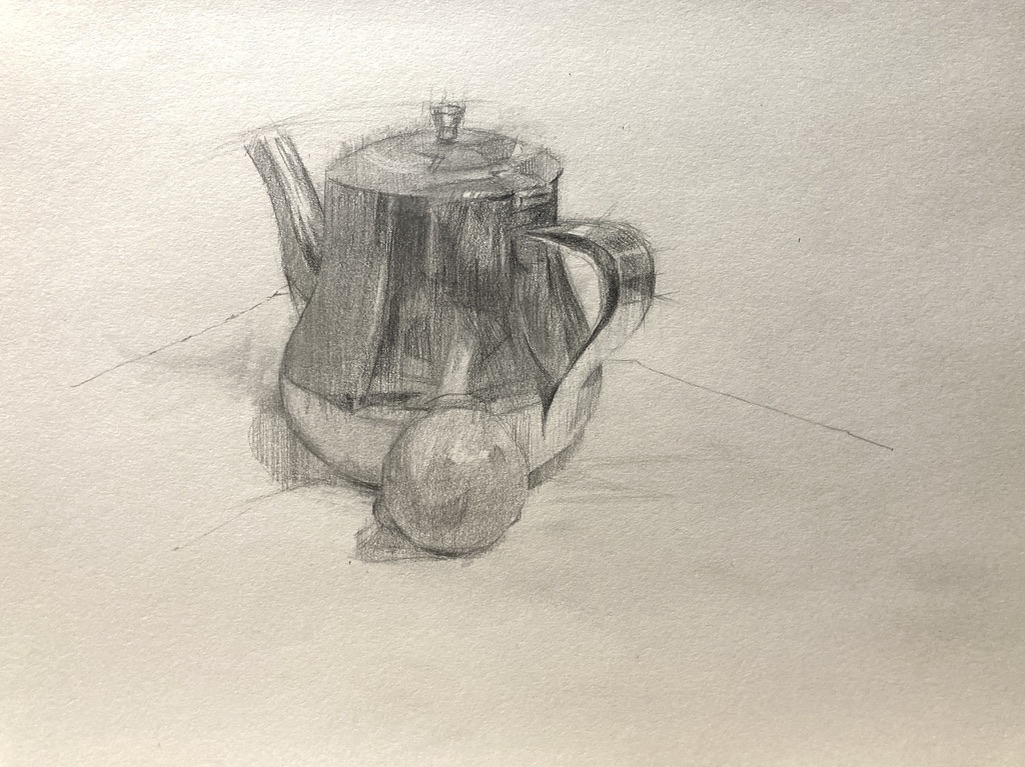A detailed hand-drawn illustration in grey pencil depicts a teapot, captured in a photograph that reveals a distinct light reflection. The bright highlight spans horizontally from the top left, about halfway across the image, suggesting a light source or camera flash. The rest of the paper has a muted, cream color, with subtle variations in shade, being lighter at the bottom left and along the vertical left edge. The teapot is shown in a near side view, with the handle positioned diagonally downward at the four o'clock position and the spout pointing outward at the ten o'clock position. The lid is securely in place, topped with an upside-down cone shape that flares outwards, likely designed for easy grasping. The teapot features a wider base that tapers slightly toward the top, where it has been shaded darker around most of its circumference. A lighter band encircles the bottom, giving the illustration the semblance of a stainless steel texture despite being sketched by hand.